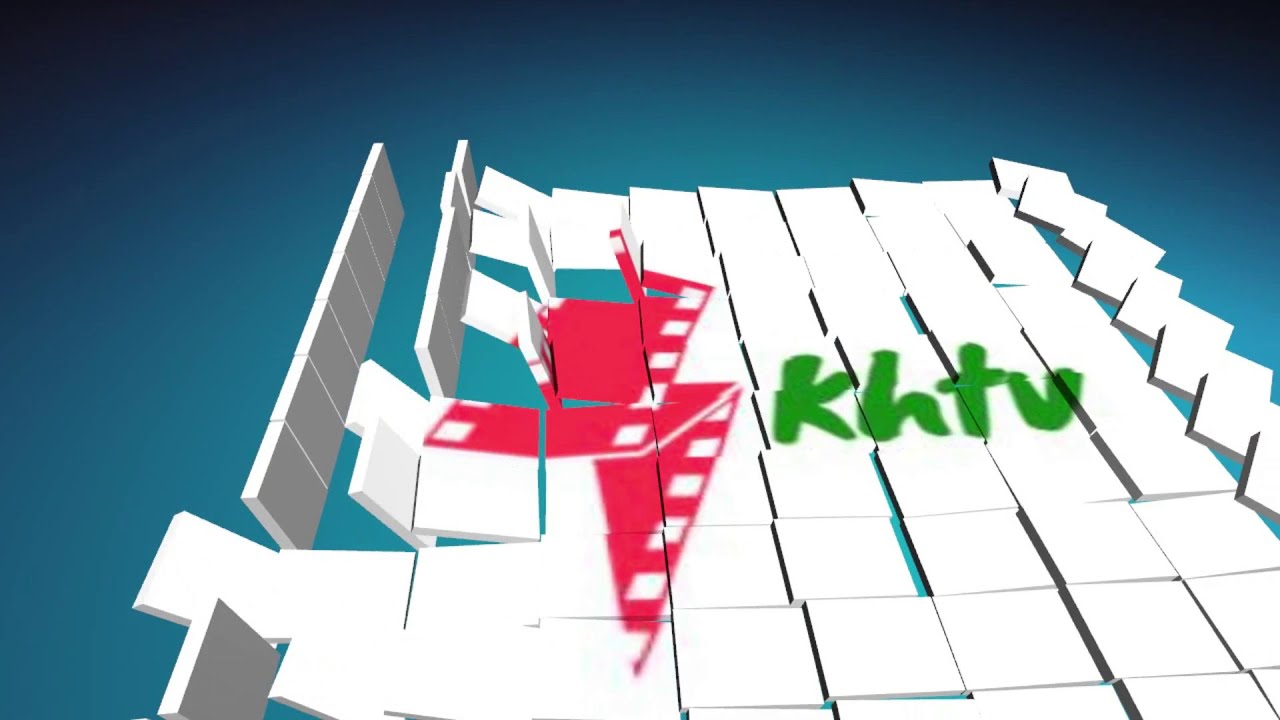The horizontal, computer-generated image features a dynamic array of white tiles against a radiant blue background that transitions from dark blue in the corners to a lighter blue towards the center. These tiles, some of which appear to be floating away from the main structure on the right and left sides, form a platform. Prominently displayed across the center of these tiles are the bright green, almost cursive letters "KHTV," suggesting a TV advertisement or channel branding. To the left of this central text is a complex red logo resembling a folded film reel, which includes a triangular base with a rectangular fold at the top and is bordered by small white squares.